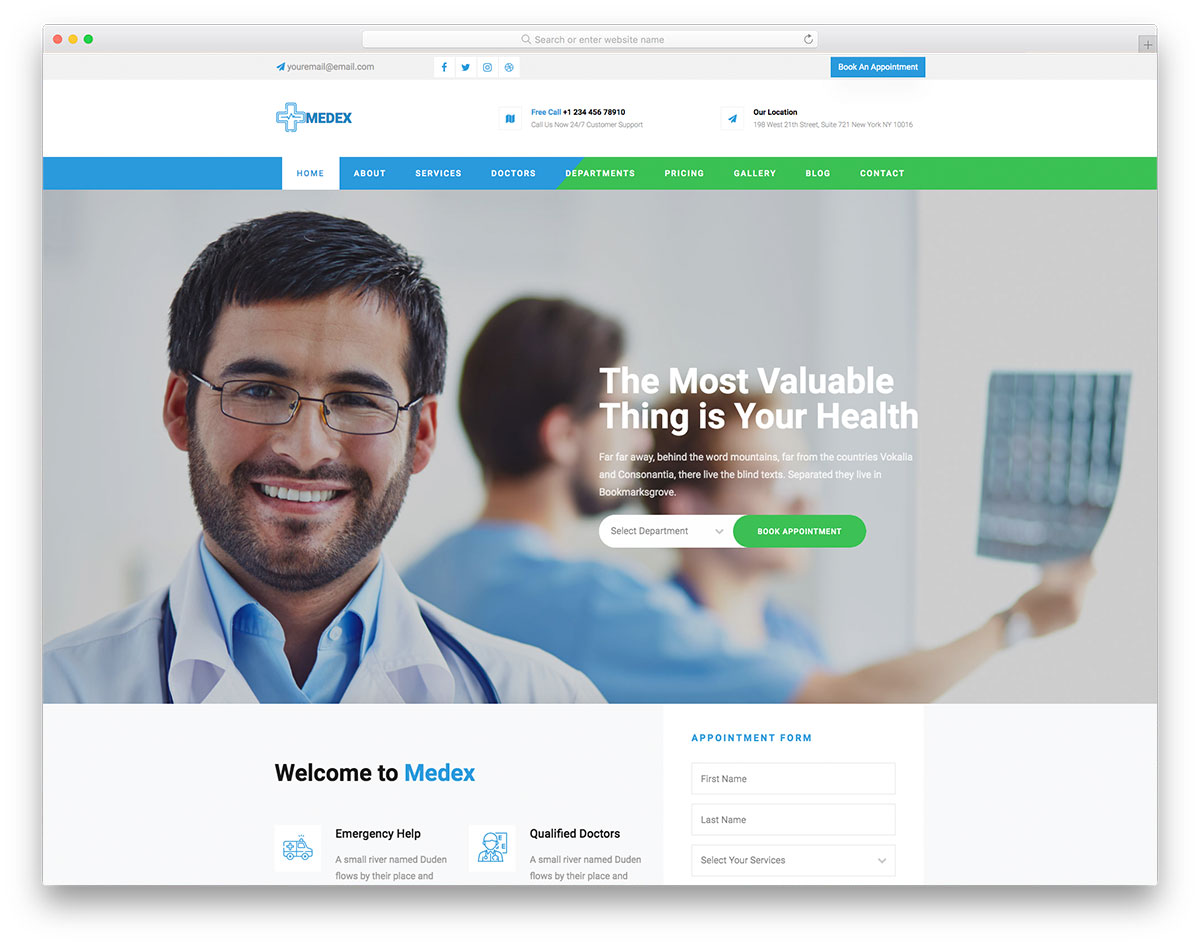**Screenshot from a Macintosh Computer**

The screenshot captures a browser window on a Macintosh computer. At the top, the dark gray bezel includes the standard close (red), minimize (orange), and maximize (green) buttons. Adjacent to these is an off-white search bar with a gray magnifying glass icon and placeholder text, "Search or enter website name." A refresh symbol sits on the right of the search bar. At the far end of the bezel is a small dark gray square with a black 'X'.

Below this, a mid-gray rectangle displays a dark blue paper airplane icon next to the text "your-email@gmail.com" in dark gray. Multiple white squares, divided by blue lines, contain various icons: a blue Facebook logo, a blue Twitter logo, a blue Instagram logo, and an icon resembling a soccer ball or a globe, possibly indicating a web browser.

On the far right is a dark blue rectangle with bold white text that reads, "Book an Appointment." Beneath this is a white rectangle containing a blue cross with a heartbeat graph and the bold, all-caps text "MedX" in dark blue. To the right is a small square with a thin gray border and a blue map icon. Next to it in cyan blue text, it says "Free Call," and in bold black it lists the phone number "+1 234-456-78910." Below, in gray text, it states, "Call us now 24-7 customer support." Another section to the right shows a dark blue paper airplane icon within a dark gray-bordered square followed by the bold black text "Our Location." Below this, in dark gray, it provides the address, "198 West 25th Street, Suite 721, New York, NY 10016."

The main visual features a smiling man in the foreground with black hair, a trimmed beard, and wearing spectacles. He sports a light blue undershirt under a white doctor's jacket and a dark blue stethoscope. In the background, another man and a woman, both in blue scrubs, examine a dark blue x-ray. The man has dark black hair and a black beard, while the woman, who wears glasses and has short blonde-brown hair, has her face slightly blurred.

At the bottom of the webpage, within a white bezel, bold black text reads, "Welcome to," followed by bold blue "Med-X." To the right, a dark blue ambulance icon is labeled "Emergency Help." Below this, in smaller black text, it states, "A small river named Duden flows by their place." Adjacent to this is a doodle of a doctor with a clock and part of the phrase "Qualified Doctors." Completing the screen, a white rectangle with cyan blue text reads "Appointment Form," containing input fields for "First Name," "Last Name," and a drop-down menu for "Select Your Services."